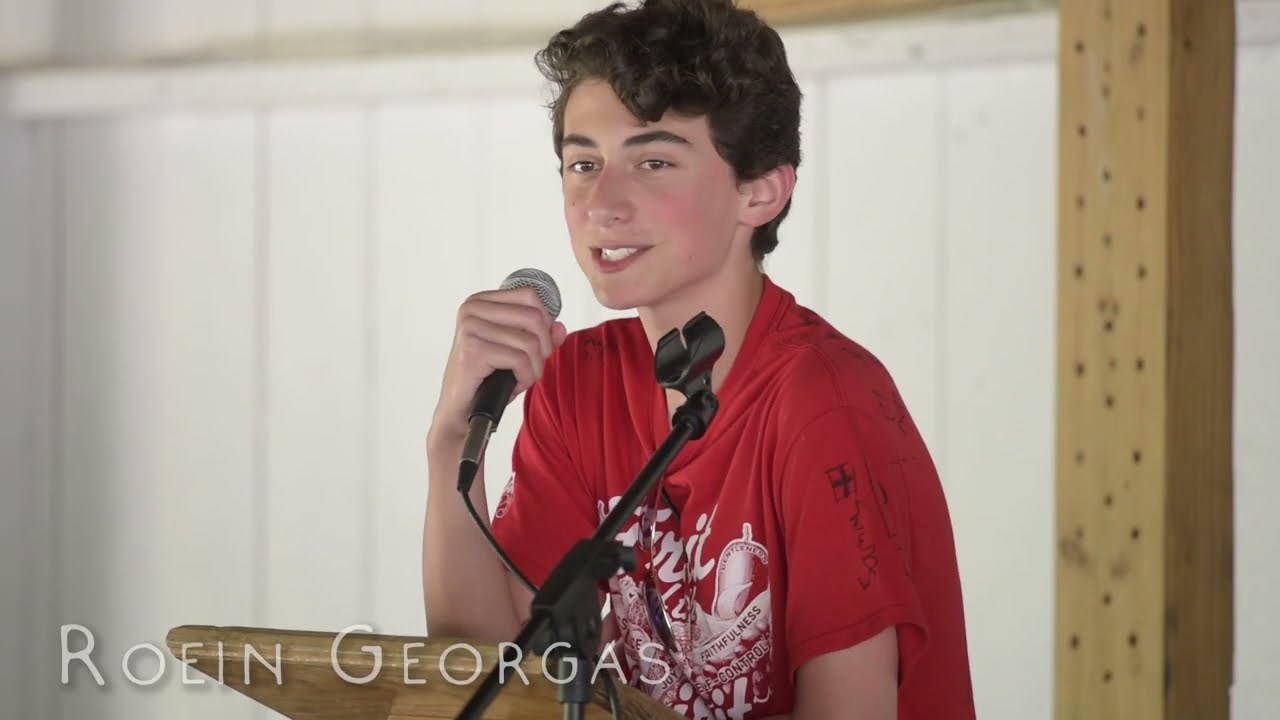This photo depicts a teenage Caucasian boy with short, curly brown hair standing at a wooden podium, delivering a speech in an outdoor pavilion with white tin walls and exposed wooden beams. Behind him, part of a wooden beam can be seen, resembling a cross. The boy is holding a microphone in his right hand, taken off the stand which is positioned to his left. He is dressed in a red T-shirt featuring a white design with words that seem to include "joy," "faithfulness," and "self-control," suggestive of the "fruits of the spirit." Signatures can be seen on his left shoulder and the back of his shirt. His mouth is slightly open, showing his teeth as he speaks, and in the bottom left-hand corner of the image, the text "Roane Georges" is visible in white type.